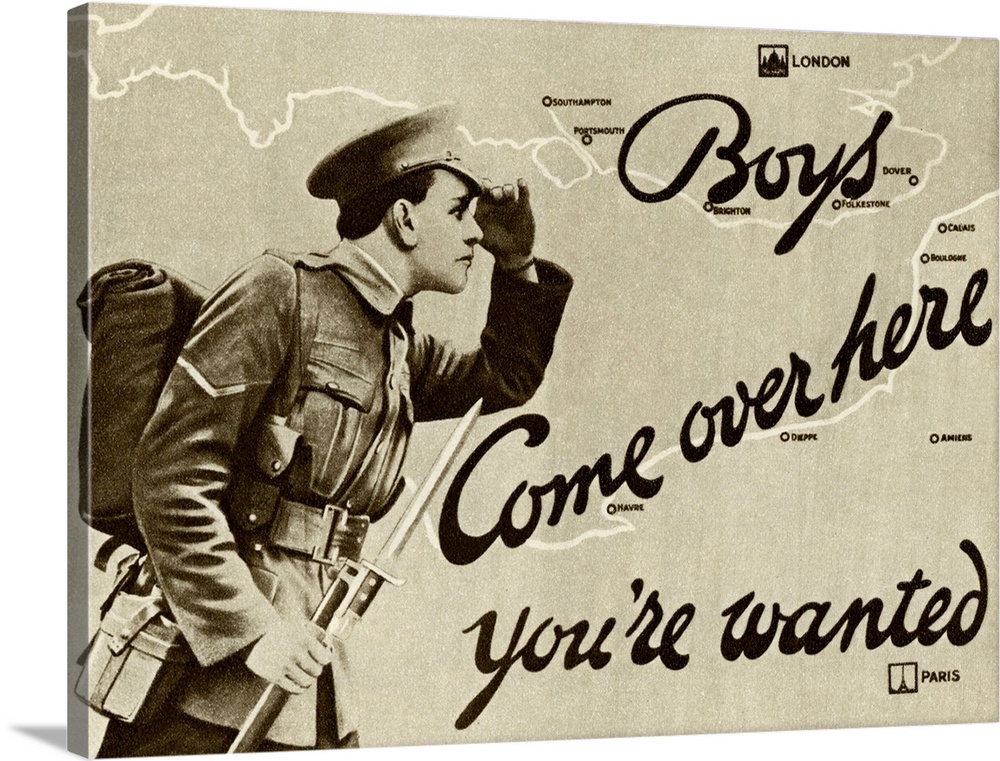This image is a vintage World War II British Army recruitment poster. Dominating the background is a detailed map showcasing the area between London and Paris, with both cities prominently highlighted using distinct icons. Additional important locations such as Southampton, Portsmouth, Brighton, Folkestone, Dover, Boulogne, Dieppe, Amiens, Havre, and Calais are also marked. On the left of the poster is an illustration of a young soldier dressed in full military uniform, complete with a cap and rifle, the bayonet visible but the lower part of the gun obscured. The soldier is depicted shielding his eyes from the sun, gazing earnestly towards the Channel. The poster's text, "Boys, come over here, you're wanted," suggests the British Army's urgent call for enlistment, likely after the fall of Paris. The background features a weathered, grayish tone, adding to the vintage feel of the image, which also appears to be transferred onto a canvas that wraps around the edges, enhancing its historical and collectible appeal.